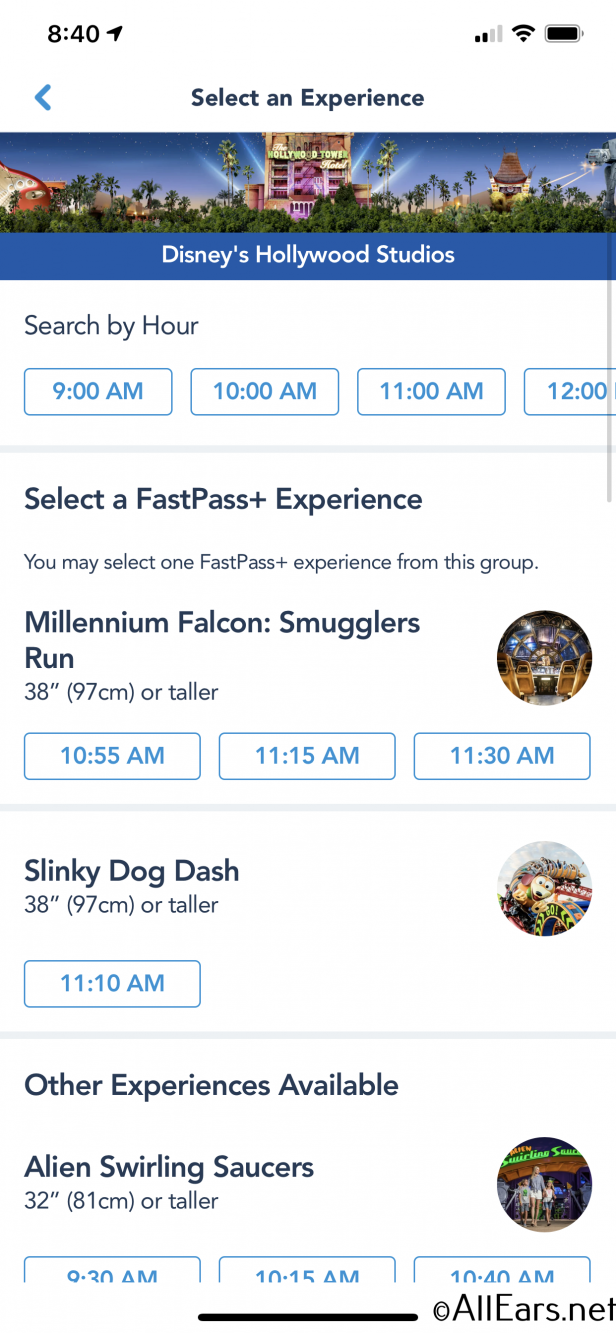The screenshot displays the interface of a mobile app designed for booking FastPass+ experiences at Disney's Hollywood Studios. At the top of the screen, a blue banner features an image of Disney's Hollywood Tower framed by palm trees. Below the image, a toolbar reads "Search by Hour" with selectable time slots, such as 9 a.m., 10 a.m., 11 a.m., and 12 p.m.

The main section of the screenshot is titled "Select a FastPass+ Experience." It specifies that only one FastPass+ can be chosen from the listed options. The first option is "Millennium Falcon: Smugglers Run," which has a height requirement of 38 inches (97 centimeters) or taller. Available time slots for this ride are 10:55 a.m., 11:15 a.m., and 11:30 a.m.

The second option listed is "Slinky Dog Dash," also requiring guests to be 38 inches or taller, with a booking time of 11:10 a.m.

Additional experiences are categorized under "Other Experiences Available." This includes "Alien Swirling Saucers," which has a height requirement of 32 inches. Available times for this ride are 9:30 a.m., 10:15 a.m., and 10:40 a.m.

In the bottom right-hand corner, the screen displays the copyright information: "Copyright © AllEars.net."